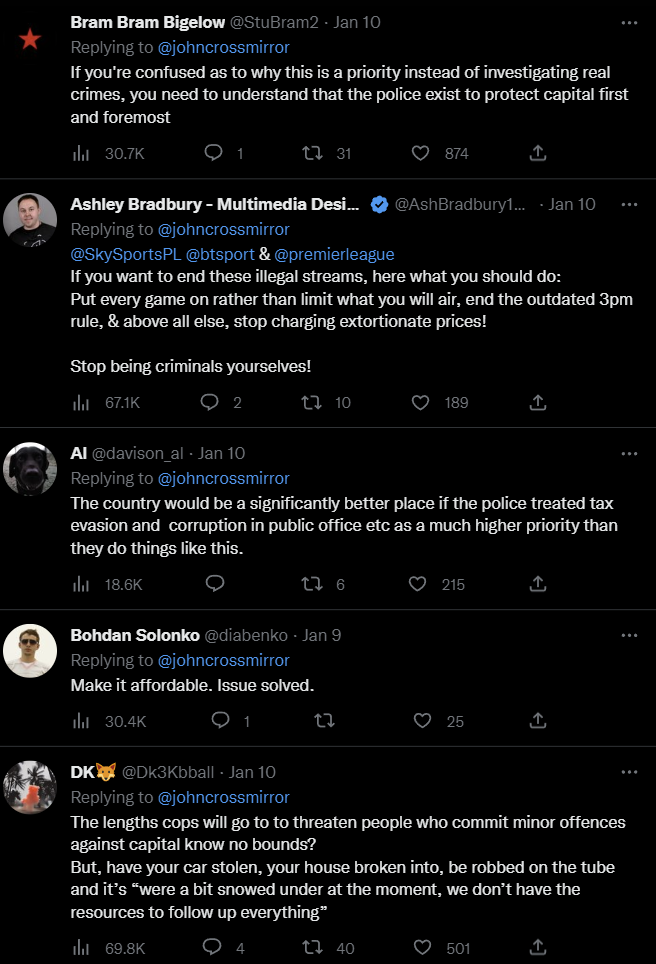***Screenshot Description: Tablet Display of Social Media Posts Related to Policing Priorities***

This image is a screenshot captured on a mobile device, likely a tablet given its moderately wide screen. The display is in portrait orientation with a black background, making the white text stand out prominently. The image appears to show a series of social media posts, possibly from Twitter given the format and the use of "@" to denote usernames.

**Post 1:**
- **Profile Photo:** Red star placeholder
- **Name:** Bram Bigelow (in bold white text)
- **Username:** @StuBram2
- **Timestamp:** Jan 10
- **Replying to:** @JohnCrossMinor
- **Content:** "If you're confused as to why this is a priority, instead of investigating real crimes, you need to understand that the police exist to protect capital first and foremost."
- **Engagement:** 
  - 30.7K views 
  - 1 comment
  - 31 reposts
  - 874 likes
  - Upload button present

**Post 2:**
- **Profile Photo:** Image of a white male (unclear age)
- **Name:** Ashley Bradbury 
- **Occupation:** Multimedia Designer
- **Content:** "If you want to end these illegal streams, here's what you should do, put every game on, rather than limit what you will air, and the outdated 3pm rule, and above all else, stop charging extortionate prices. Stop being criminals yourselves."
- **Engagement:** Standard social media statistics (likes, comments, reposts) presented under the post but unspecified in the caption.

**Post 3:**
- **Profile Photo:** Black and white photo of a dog
- **Username:** AI
- **Content:** "The country would be a significantly better place if the police treated tax evasion and corruption in public office, etc., as a much higher priority than they do things like this."

**Post 4:**
- **Profile Photo:** A person with glasses on a white circle background
- **Name:** Bodon Solonco
- **Content:** "Make it affordable, issue solved."

**Post 5:**
- **Profile Photo:** Unclear, possibly a fox or cat emoji
- **Username:** DK
- **Content:** "The lengths cops will go to threaten people who commit minor offenses against capital know no bounds, but have your car stolen, your house broken into, be robbed on the tube, and it's, we're a bit snowed under at the moment, we don't have the resources to follow up everything."

Each post reflects a critical stance on policing priorities, highlighting a common theme of dissatisfaction with law enforcement's focus on protecting capital over addressing what these users consider more significant crimes.